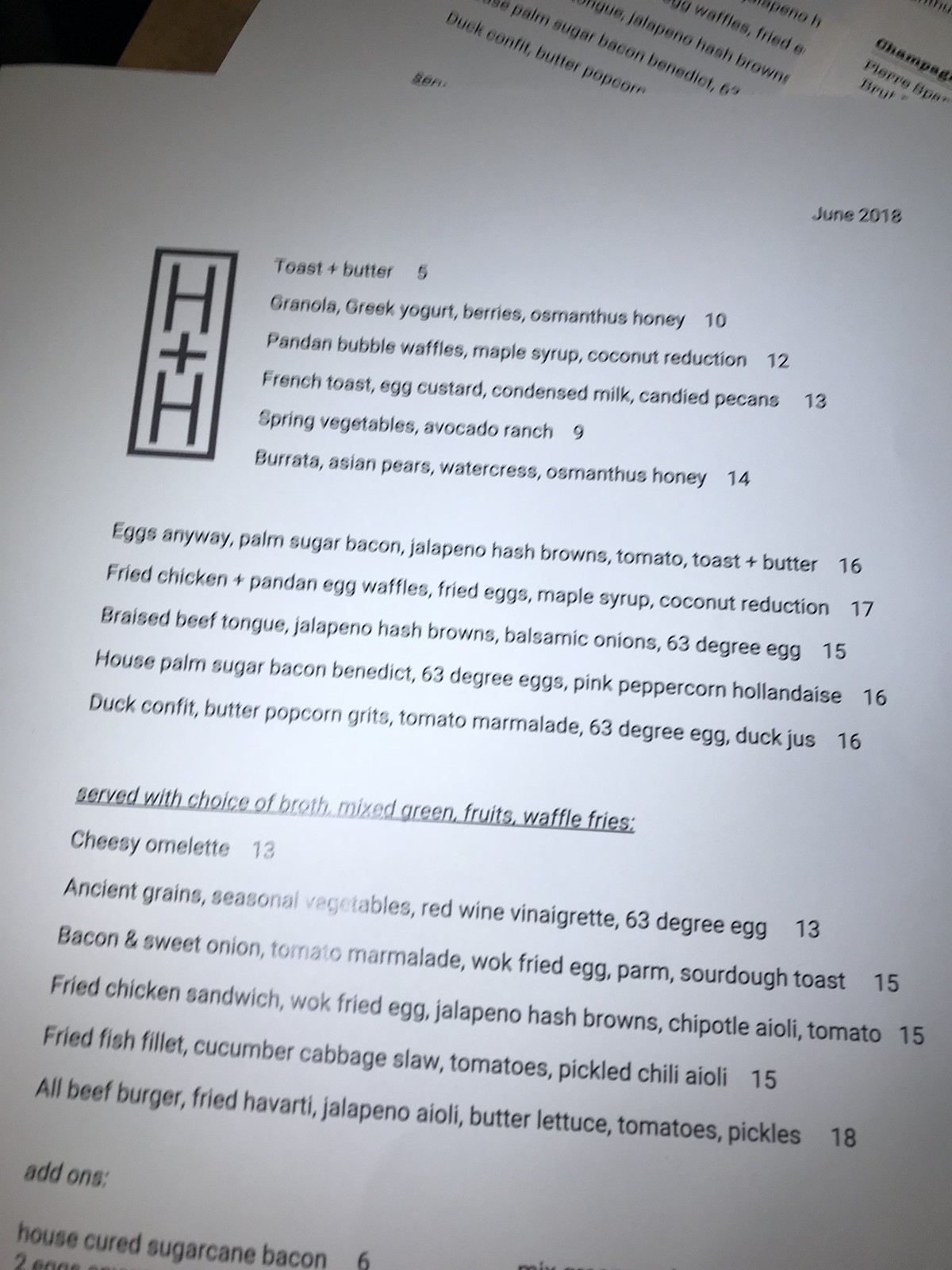A detailed caption for the image could be:

The image showcases a white menu, either a paper or laminated sheet, placed on a flat surface. Another similar white menu is partially visible beneath it. The menu features the restaurant logo, "H+H," where "H" is stacked above a "plus" sign, which is followed by another "H." In the top right corner, the menu is dated "June 2018." 

The menu lists a variety of items with their prices:

1. **Toast + Butter**: $5
2. **Granola, Greek Yogurt, Berries, Osmanthus Honey**: $10
3. **Pandan Bubble Waffles, Maple Syrup, Coconut Reduction**: $12
4. **French Toast, Egg Custard, Condensed Milk, Candied Pecans**: $13
5. **Spring Vegetables, Avocado, Ranch**: $9
6. **Burrata, Asian Pears, Watercress, Osmanthus Honey**: $14

Following this, the items are aligned under the "H+H" logo:

1. **Eggs Anyway, Palm Sugar Bacon, Jalapeno Hash Browns, Tomato, Toast + Butter**: $16
2. **Fried Chicken, Pandan Egg Waffles, Fried Eggs, Maple Syrup, Coconut Reduction**: $17
3. **Braised Beef Tongue, Jalapeno Hash Browns, Balsamic Onions, 63 Degree Egg**: $15
4. **House Palm Sugar Bacon Benedict, 63 Degree Eggs, Pink Peppercorn Hollandaise**: $16
5. **Duck Confit, Butter Popcorn Grits, Tomato Marmalade, 63 Degree Egg, Duck Jus**: $16

A section indicates the items are served with a choice of broth, mixed greens, fruits, or waffle fries. The following items are listed:

1. **Cheesy Omelet**: $13
2. **Ancient Grains, Seasonal Vegetables, Red Wine Vinaigrette, 63 Degree Egg**: $13
3. **Bacon and Sweet Onion, Tomato Marmalade, Wok Fried Egg, Palm, Sourdough Toast**: $15
4. **Fried Chicken Sandwich, Wok Fried Egg, Jalapeno Hash Browns, Chipotle Aioli, Tomato**: $15
5. **Fried Fish Fillet, Cucumber, Cabbage Slaw, Tomatoes, Pickle, Chili Aioli**: $15
6. **All Beef Burger, Fried Havarti, Jalapeno Aioli, Butter Lettuce, Tomatoes, Pickles**: $18

At the bottom corner, there's a section for add-ons, listing items such as house-cured sugarcane bacon ($6), and partially visible two eggs with an incomplete description.